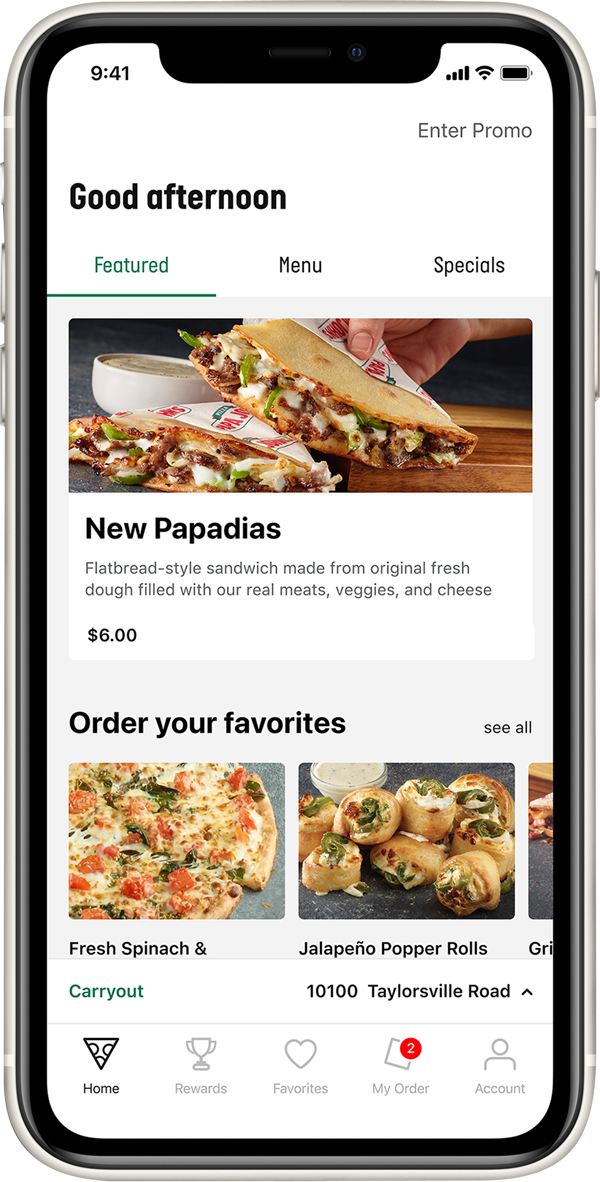This illustration features a detailed depiction of a white cell phone with a black outline. The phone's screen has a predominantly white background. In the upper left corner of the screen, the time "9:41" is displayed. The upper right corner shows signal indicators for service bars, Wi-Fi, and battery life.

Beneath these indicators, in black lettering, the left side reads "Good afternoon" while the right prompts "Enter promo." Below this greeting, there are three selectable tabs: "Featured" on the left, "Menu" in the center, and "Specials" on the right.

A prominent image showcases a food item labeled "Papadias" with a description stating "New Papadias Flatbread-style sandwich made from original fresh dough filled with our real meats, veggies, and cheese - $6." Below this, an invitation reads "Order your favorites" followed by "See all."

The screen also displays images of various meals, including a pizza topped with fresh spinach and a tray of jalapeño popper rolls. Below these meal options, the text "Carry Out" appears in blue lettering. 

The address "10100 Taylorsville Road" is listed on the right side, presumably the user's address. At the bottom of the screen, there are five navigation options represented by icons: "Home" with a pizza symbol, "Rewards" with a trophy, "Favorites" with a heart, "My Order" with a box, and "Account" at the end.